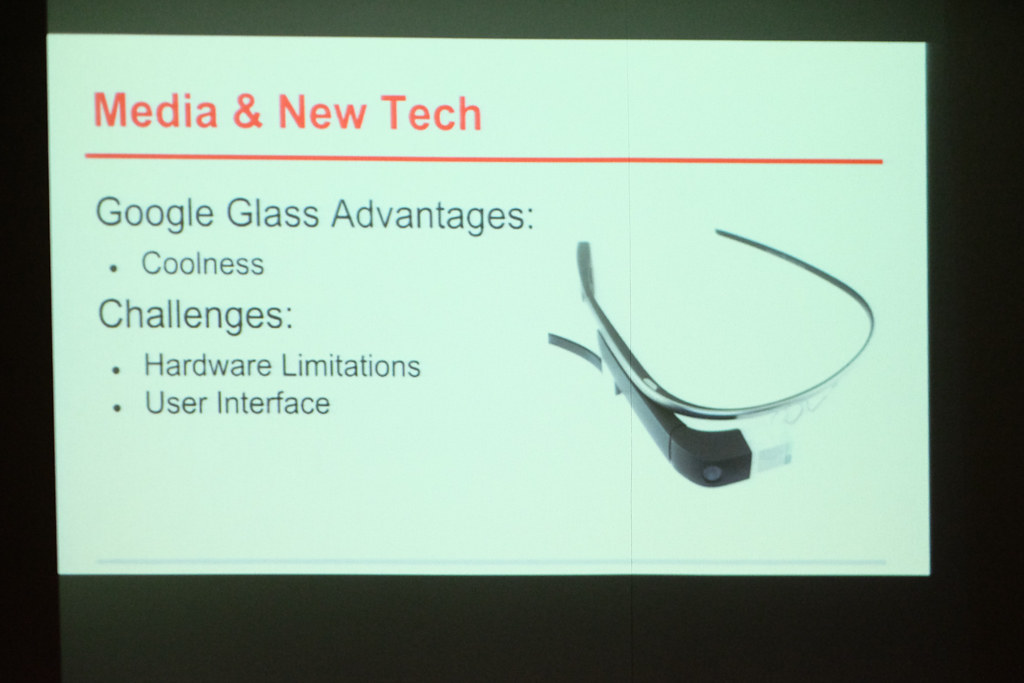This image captures a slide from a PowerPoint presentation set against a primarily black background with accents of green at the top and bottom. Central to the slide is a depiction of a computer screen displaying a white background. Dominating the top of the screen, the title "Media and New Tech" is prominently showcased in bold red letters, underneath which a solid red horizontal line stretches across the width of the image. Below this line, the content is divided into two categories: "Google Glass Advantages" and "Challenges," both in black text. Under "Google Glass Advantages," the bullet point "coolness" is noted. The "Challenges" category lists "hardware limitations" and "user interface" issues. On the right side of the image, there is a visual representation of Google Glass, resembling headphones with a distinctive semicircle shape. This slide provides an overview of Google Glass, an early AR device that paved the way for contemporary VR and AR technologies, outlining both its potential benefits and its limitations.